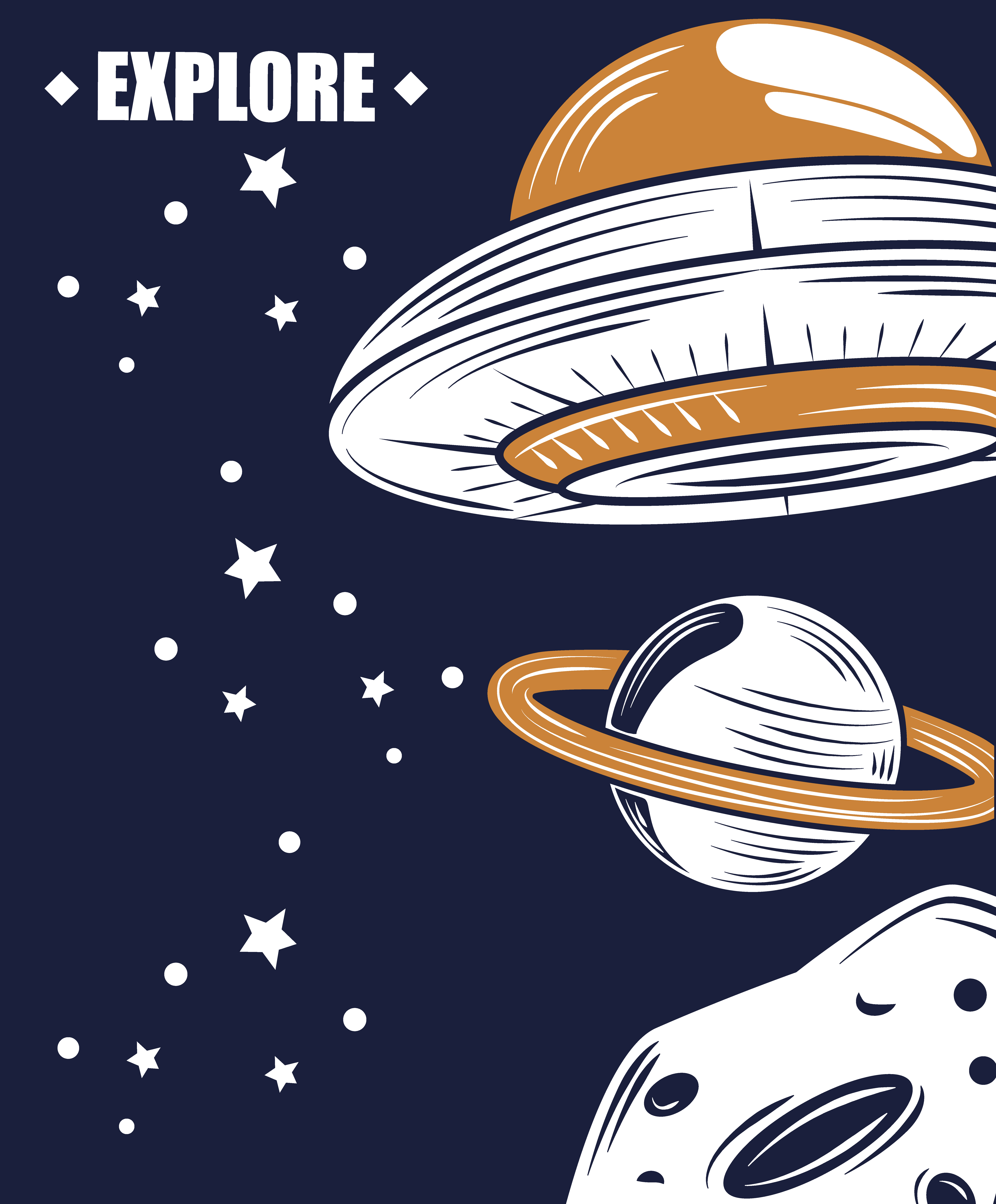The image is a simplistic, two-color space-style poster with a portrait orientation and a rectangular shape, with the height being twice the length of the width. The background is predominantly dark blue. In the top left corner, the word "EXPLORE" is displayed in large, bold, white capital letters, flanked by small white diamond shapes on either side. Cascading below "EXPLORE" are an array of white five-pointed stars and white circles, arranged vertically along the left side. On the right side of the poster, a large alien saucer with an orange, dome-shaped top and a white rim occupies the top right corner, angled slightly toward the center. Below the saucer is a white planet with an orange ring, resembling Saturn, which is tilted slightly. In the very bottom right corner, there is a partially visible white asteroid with blue circles, suggesting craters.